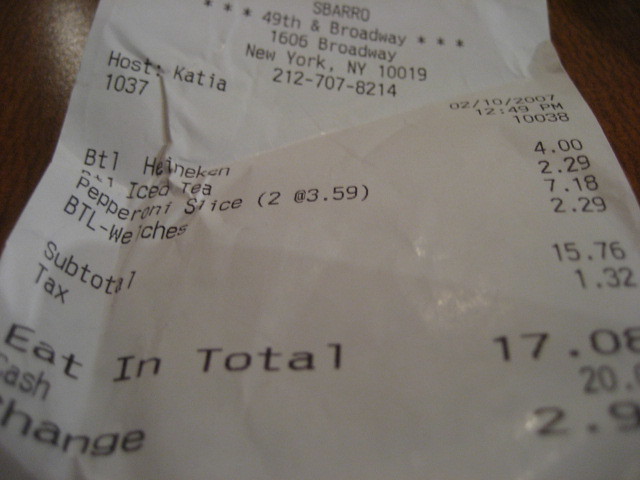In this image, we see a close-up shot of a receipt from the restaurant Sbarro, placed on a brown table surface. The background of the receipt shows a bit of white light reflecting on the top left corner. 

At the very top of the receipt, the restaurant name "Sbarro" is prominently printed. Just below the name, the address "49th and Broadway" is flanked by three stars on both the left and right sides. Further down, the full address "1606 Broadway, New York, NY 10019" is listed along with a phone number.

The receipt details include the host's name on the left and the date, time, and zip code on the right. The ordered items follow, including a "Heineken," "iced tea," "pepperoni slice," and "BTL Welch's." The prices for each item are aligned on the right-hand side of the receipt.

Towards the bottom, the subtotal is noted as $15.76, with a tax amount of $1.32. The total amount due is prominently displayed as $17.08. The receipt itself is light gray with black text, making the details easily readable.